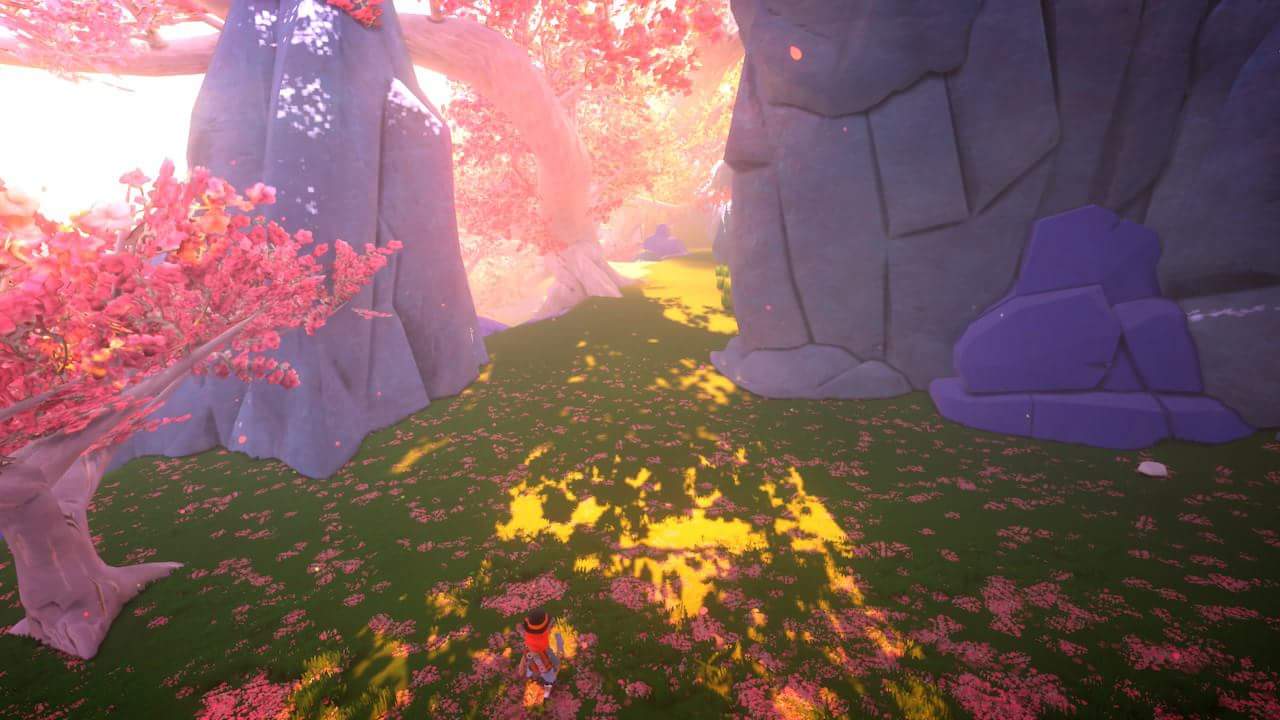In this mesmerizing fantasy landscape, the foreground features a dark, almost black terrain splattered with vibrant purple and yellow paint. Resting on this peculiar ground is an enigmatic red object, adorned with a black circle and encircled by a black ring. Toward the back, a captivating opening reveals a forest of otherworldly purple trees, their yellow leaves contrasting sharply with the surrounding darkness. This entrance is framed by a collection of large, cobbled purple stones that add to the scene's mystical atmosphere. To the left, a striking purple tree with leaves in shades of pink, orange, and a hint of yellow stands tall against the black and purple-spattered ground, enhancing the fantastical essence of this enchanted setting.